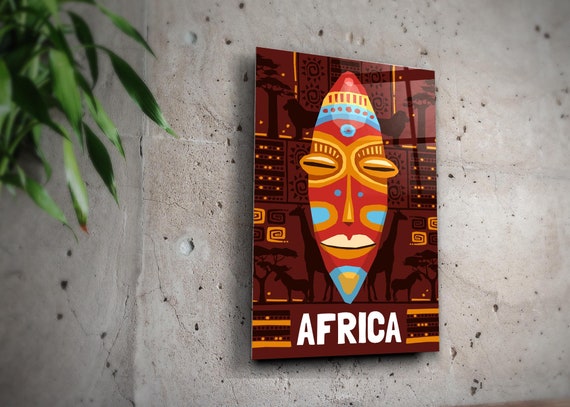The image features a detailed and textured gray stone wall adorned with numerous tiny circular holes, providing a rugged backdrop. In the upper left corner, green leaves from a plant cascade down into the frame. Affixed to the wall and prominently displayed is a rectangular brown poster that captures the viewer's focus. The poster showcases a vibrant tribal mask adorned with striking red, yellow, blue, and cream colors. The mask features prominent buggy eyes, a thin nose, and a detailed chin. Surrounding the mask are silhouettes of African animals like giraffes and lions against the brown background. At the bottom center of the poster, the word "AFRICA" stands out in large white capital letters, flanked by yellow and brown stripes with dots. This work of art evokes the rich cultural heritage and natural beauty of Africa.